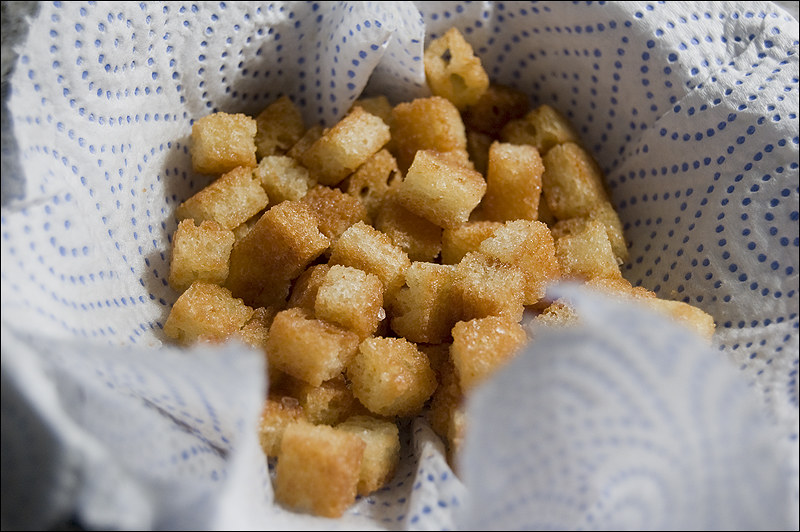The image features a bowl-shaped basket lined with a white paper towel that has a blue dotted, swirled pattern. The paper towel extends slightly over the edges of the basket. Inside the basket are about 30 to 35 small, golden-brown, cube-shaped croutons. They appear lightly oily, with a crisp, darker brown top surface. The image is closely zoomed in, bringing detailed focus to the croutons and their texture. The background does not display any other elements, emphasizing the contents of the basket. Light seems to be coming from above, casting subtle shadows and highlighting the colors and textures of both the croutons and the patterned paper towel.